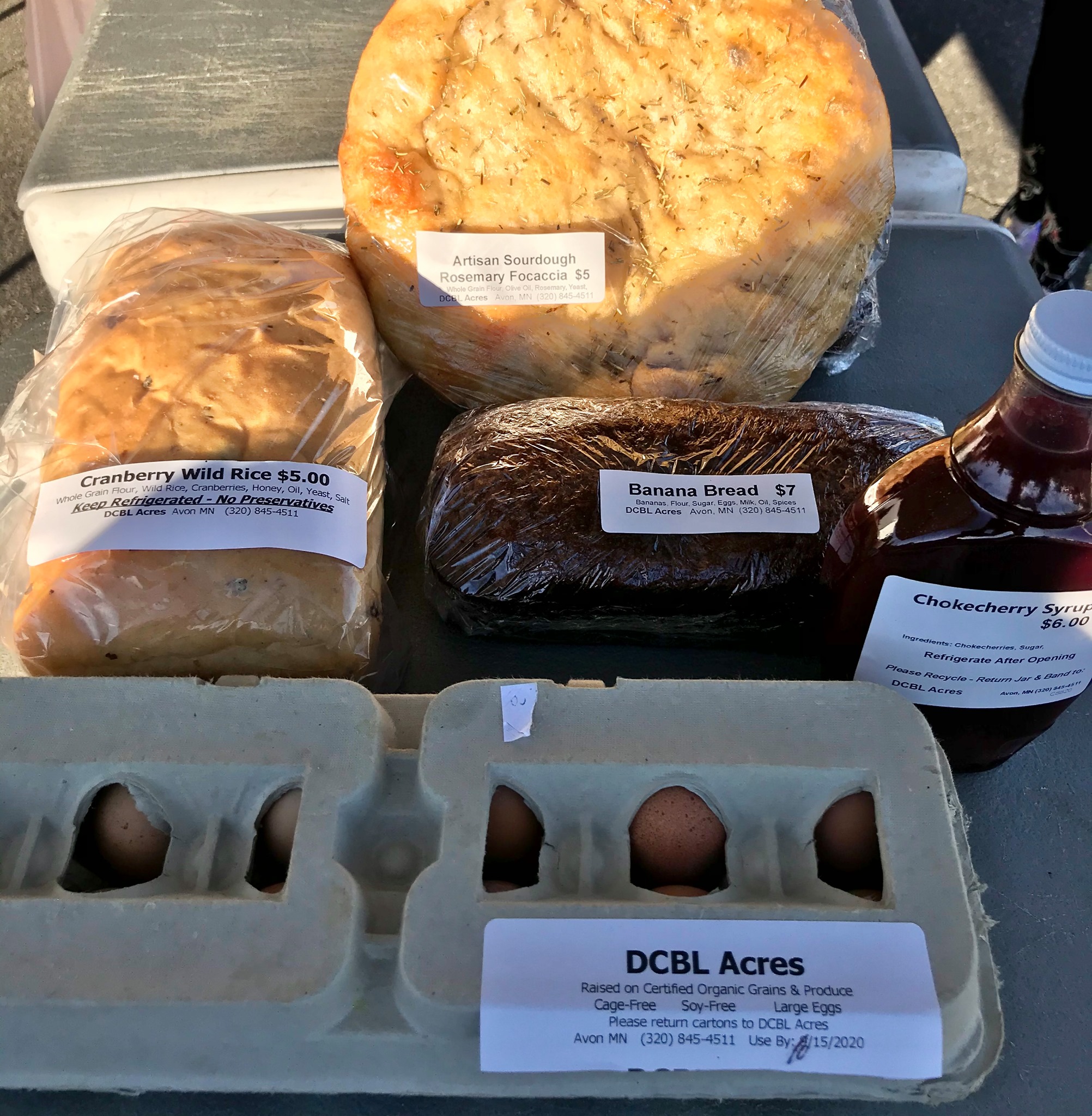The vertical rectangular image showcases an assortment of items for sale at a farmer's market, meticulously arranged on a table. Prominent in the foreground is a gray cardboard carton of brown eggs, marked with a white label reading "DCBL Acres," indicating their source. Detailed text on the label mentions they are raised on certified organic grains and produce, cage-free, soy-free, and large, with a request to return the cartons to DCBL Acres. Behind the carton, three distinct loaves of bread are lined up: a dark loaf identified as Banana Bread with a price tag of $7, a lighter loaf labeled Cranberry Wild Rice priced at $5, and a round loaf labeled Artisan Sourdough Rosemary Focaccia with a price of $3. Additionally, to the right, a bottle with a red liquid and a white cap is labeled Choke Cherry Syrup, priced at $8. Each item features a simple white rectangular sticker with black text, detailing their names and prices, unifying their presentation.